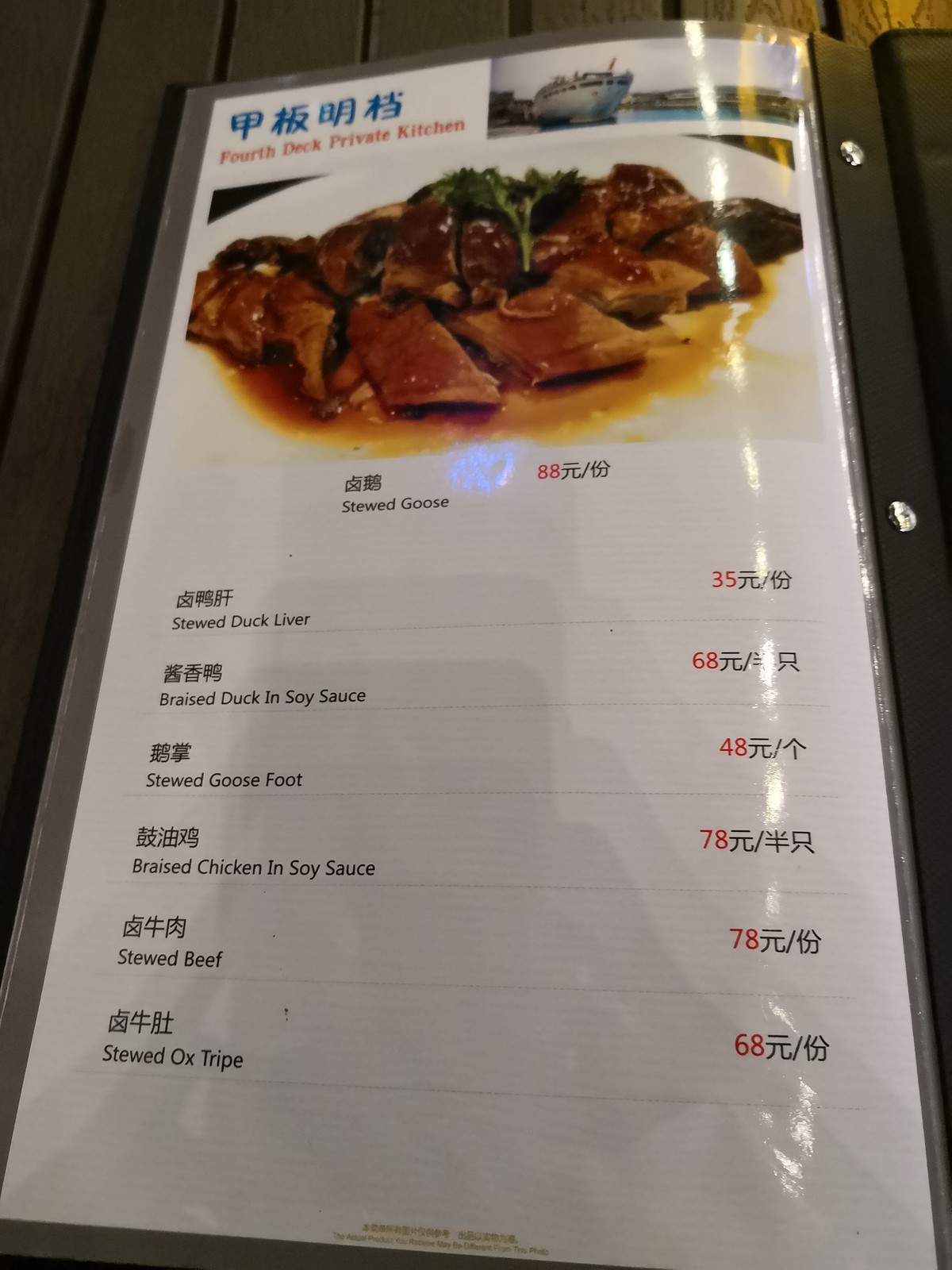The image features a detailed shot of a menu placed on a surface made of wooden slats, which are about two inches wide with a quarter-inch gap between them. The slats have a grayish-brown hue with darker streaks, suggesting a rustic, natural wood finish. While it's not entirely clear if this surface is a table, its alignment and composition suggest it could be.

The menu itself is printed on a white page and is held within a black binder. The white page is encased in a plastic sleeve and is bound at the top with at least two visible holes. The top left corner of the menu features blue Chinese lettering. Adjacent to this, in the top right corner, is an image of a boat floating on a serene body of water with hills lining the horizon.

Beneath this, there's a photograph of a plate filled with bite-sized pieces of meat coated in a rich, dark brown gravy. The dish is garnished with a sprig of parsley near its center and is presented on a white plate with a slight black rim visible at the top and right sides.

The menu lists various traditional dishes with both Chinese characters and English translations:
- Stewed Goose: $88
- Stewed Duck Liver: $35
- Braised Duck in Soy Sauce: $68
- Stewed Goose Foot: $48
- Braised Chicken in Soy Sauce: $78
- Stewed Beef: $78
- Stewed Ox Tripe: $68

At the bottom center of the menu, some additional writing is visible, although it is not detailed in the description. The overall presentation suggests a high-quality, authentic dining experience.